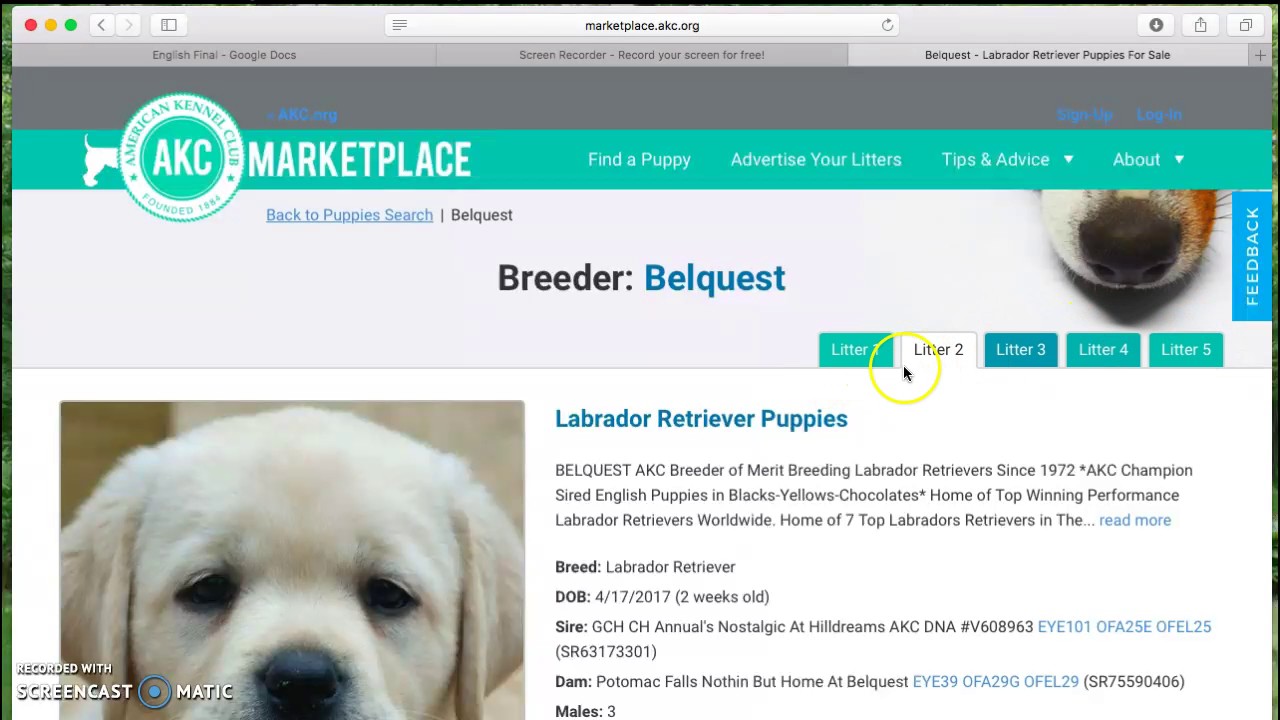**Captivating Desktop Snapshot of AKC Marketplace**

The screenshot captures a detailed view of a desktop browser opened to the American Kennel Club Marketplace website (marketplace.akc.org). The window's silver browser frame is visible at the top, featuring three colored dots on the far left—red, yellow, and green—indicative of the typical window control buttons. Adjacent to these, there are two light gray arrow buttons for navigating back and forth. Additionally, a smaller windows-control button, presumably for minimizing or maximizing the window, is displayed to the right. Centered within the browser bar is the URL, "marketplace.akc.org," typed in lowercase letters.

Below the address bar, three browser tabs are noticeable. The first tab is titled "English Final, Google Docs," the middle tab reads "Screen Recorder – Record your screen for free," and the focused tab is the AKC Marketplace webpage. The AKC Marketplace page is distinguished by a teal banner at the top, sporting the AKC logo and several navigation options—Find a Puppy, Advertise Your Litters, Tips and Advice, About—aligned to the right.

The webpage prominently features a section showcasing a breeder named "Belquest." A thick photo header partially reveals a dog's nose entering the frame from the top right, and an overlaying text label identifies the breeder, "Belquest." Further down, there's a partial but clear image of a puppy making direct eye contact with the camera. To the right of this image, the text "Labrador Retriever Puppies" appears in blue, with additional breeder information following below.

At the bottom left corner of the screen, a watermark labeled "Recorded with Screencast-O-Matic" indicates that the screen view is recorded. This meticulously detailed snapshot provides a comprehensive look at the AKC Marketplace interface as navigated by the user.